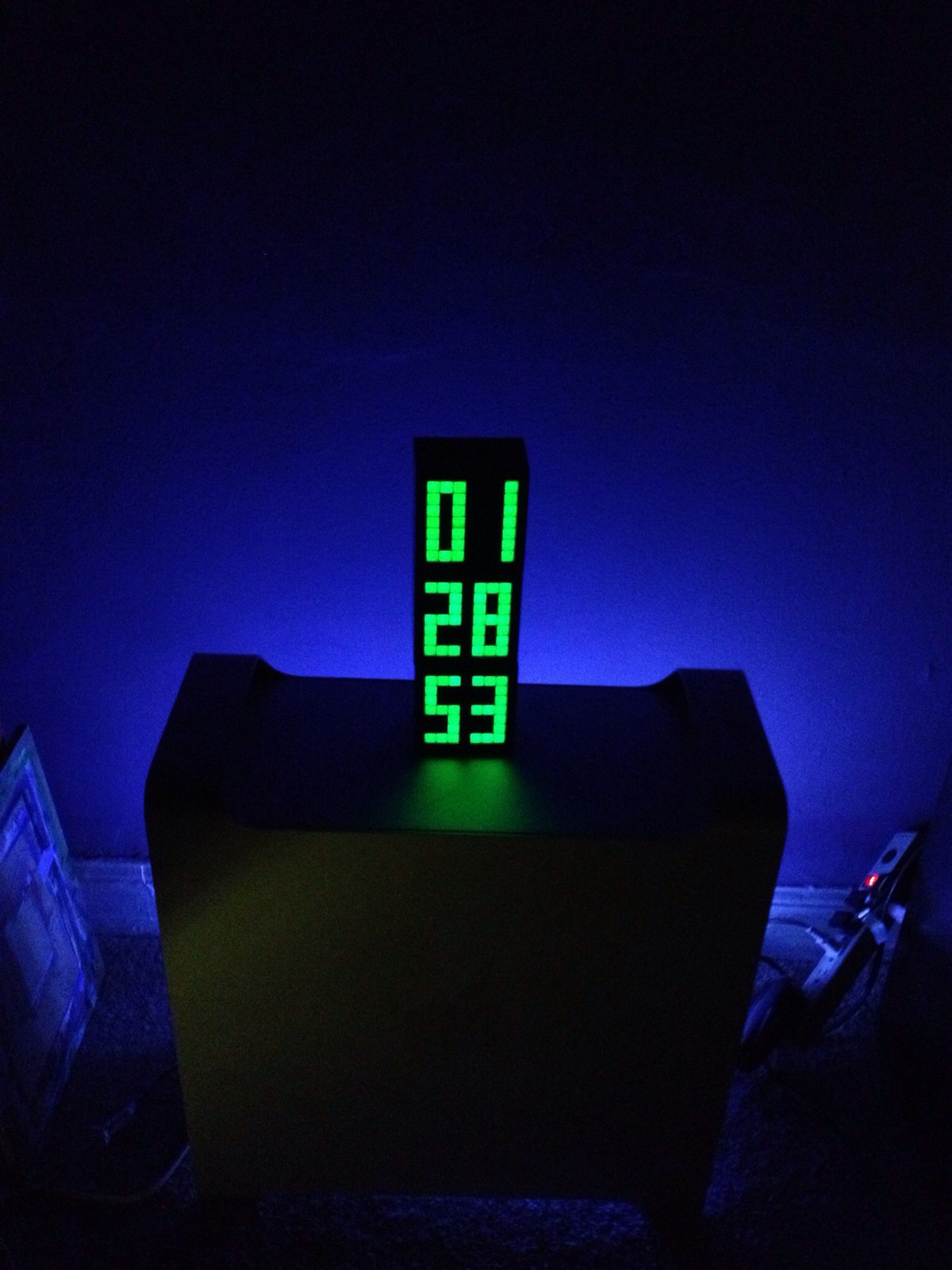This image captures a dimly-lit scene inside a piece of dark furniture that rests on the floor, shrouded in shadows. From behind the cabinet, a soft blue light emanates, casting an ethereal glow on the surrounding items and the wall. Atop the cabinet sits a digital rectangular display, illuminated with green numbers reading "01," "28," and "53" in a vertical sequence. The display, encased in a dark rectangular frame, is the focal point of the image. Flanking the cabinet on either side are partially visible electronic components, with a faint red light emanating from a component on the right, adding a subtle contrast to the overall dark ambiance. The interplay of the blue and red lights with the shadows creates a mysterious and intriguing atmosphere.